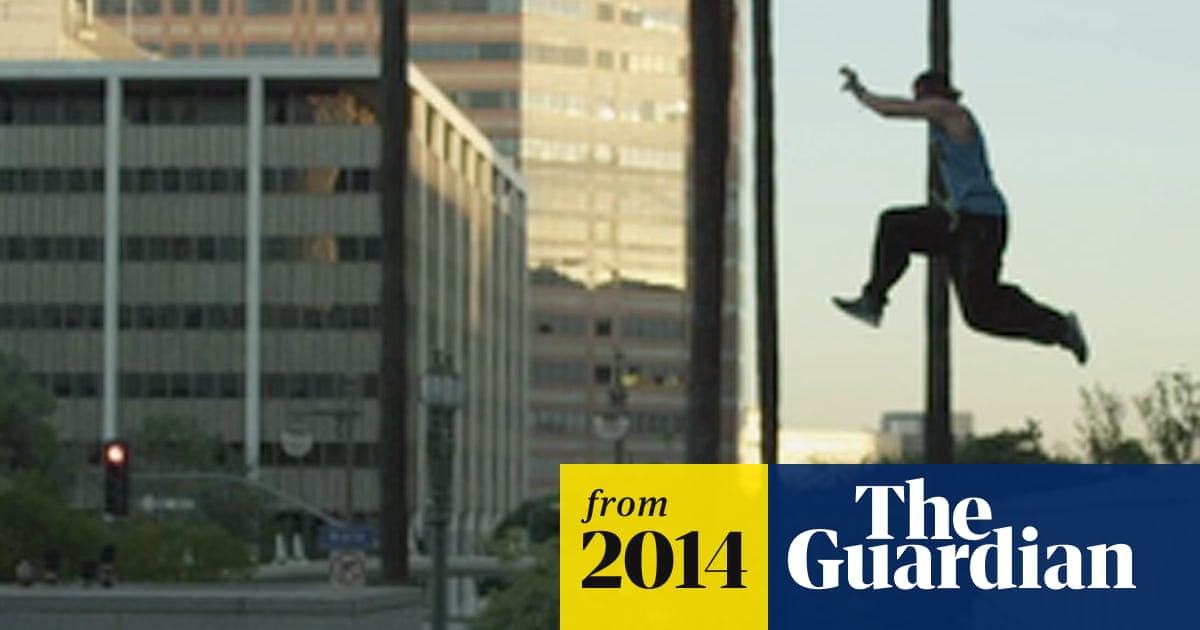In this lively cityscape photograph, a person is captured mid-air, appearing to jump across the scene, likely performing a parkour move. The individual is wearing a blue tank top, black pants, and possibly a backward hat and gloves, though the details are somewhat blurry. The backdrop features tall industrial or corporate buildings with noticeable windows, and a smaller building with some greenery and sidewalk lampposts situated in front of them. A red traffic light is visible on the street below, enhancing the urban atmosphere. The sky overhead is a clear blue, casting sunlight and shadows on the buildings. At the bottom right of the image, there is text overlaid with a yellow box that says "From 2014" in black, and a blue banner with the white text "The Guardian."